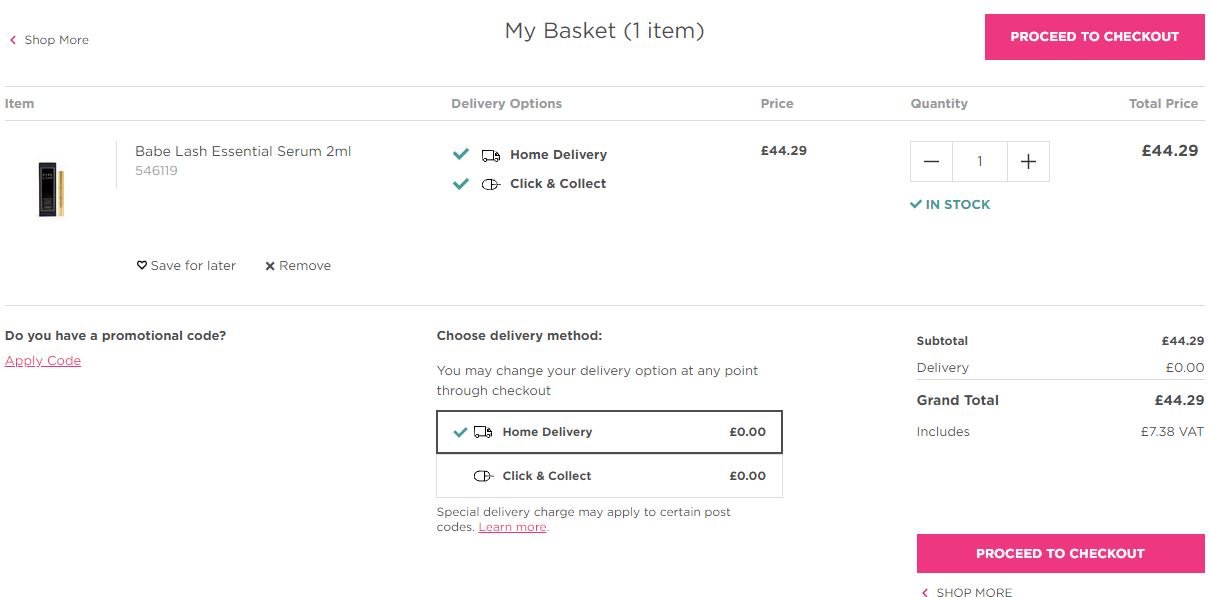This image appears to be a screenshot from a UK-based shopping website, primarily displaying a clean, white background. 

In the upper section of the screen, centered, is the heading "My Basket" in a black or dark gray font, indicating that there is one item currently in the basket. The single item listed is "Babe Lash Essential Serum, 2 milliliters," identified by the product number 546119. 

Next to this item, there are options to either save it for later, represented by a heart icon, or remove it with an X icon. The delivery options available are "Home Delivery" and "Click and Collect." 

The price of the item is 44.29 euros, with the quantity set to one. The availability is marked with a green check and the words "IN STOCK" in all caps and green color. The total price of the basket is also 44.29 euros. 

Below this section, it asks, "Do you have a promotional code?" in a black font. Adjacent to this text is a hot pink hyperlink labeled "Apply Code" with initial capitalization. 

To the right, in the same section, it prompts the user to choose a delivery method, reiterating the options: "Home Delivery" and "Click and Collect."